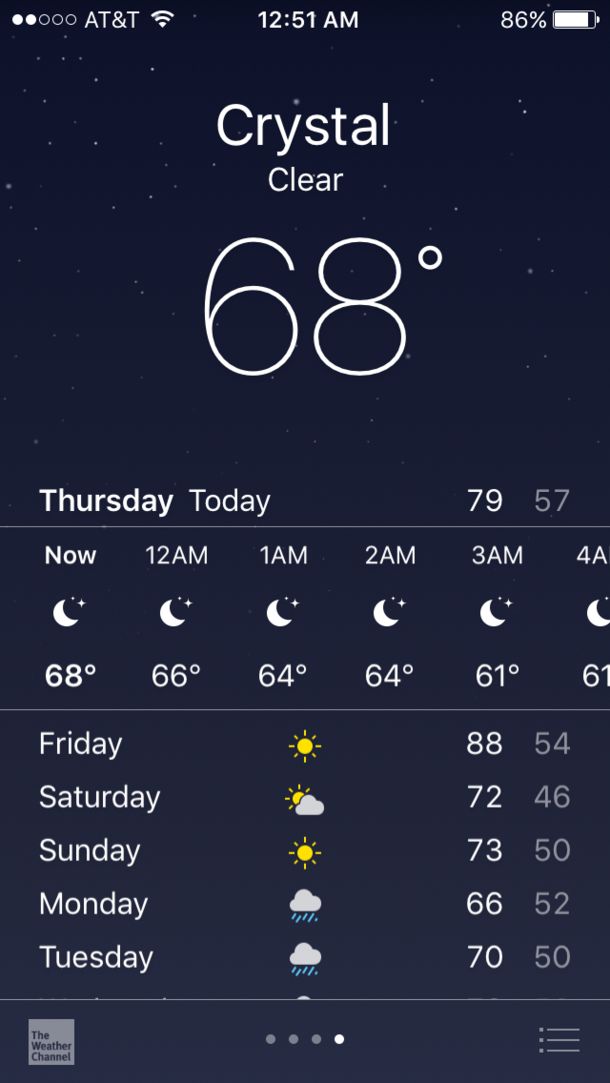This is a screenshot of a weather application displayed on a mobile phone. At the top, there is a banner containing multiple icons. From left to right, it includes two filled white circle indicators, followed by the AT&T logo, a cellular signal icon, the time (12:51 AM), and an 86% battery icon. Centered at the top, the screen displays the current weather conditions: "Crystal Clear" with a temperature of 68°F.

Below this is a chart detailing the hourly forecast for Thursday. It shows the current time, extending from now until 4 AM, with temperatures listed as 68°F, 66°F, 64°F, 64°F, 61°F, and 61°F. The temperature range for Thursday is also indicated as a high of 79°F and a low of 57°F.

Further down, a list of the weekly forecast from Friday to Thursday is presented. Each day is accompanied by a respective weather icon:
- Friday: Sunny with a high of 88°F and a low of 54°F.
- Saturday: Partially sunny with a high of 72°F and a low of 46°F.
- Sunday: Sunny with a high of 73°F and a low of 50°F.
- Monday: Rain with a high of 66°F and a low of 52°F.
- Tuesday: Rain with a high of 70°F and a low of 50°F.

The entire screenshot is set against a black background, enhancing the clarity of the displayed information.